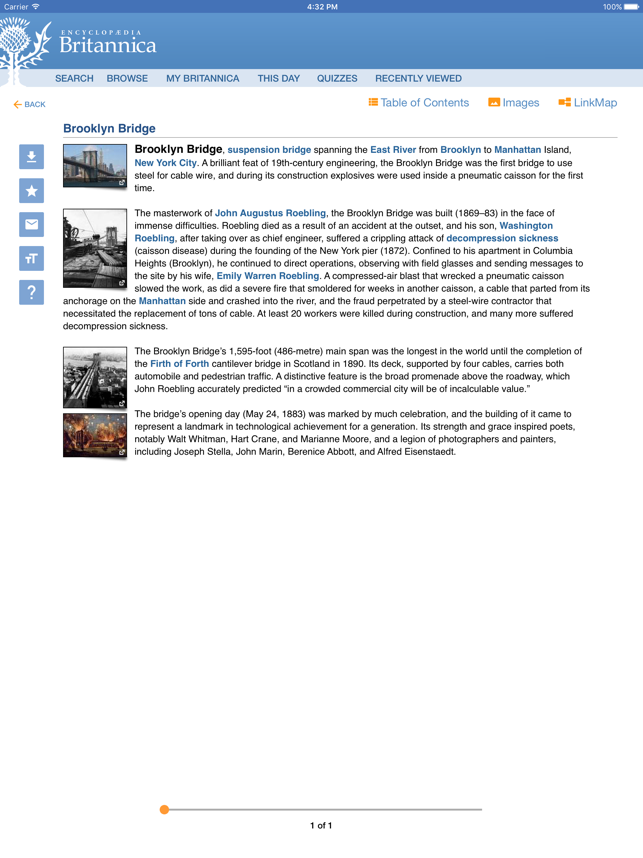The digital encyclopedia displayed on an iPad features the Encyclopedia Britannica interface, characteristic of iOS and Apple. The header displays "Encyclopedia Britannica" in white text on a blue background, with a white logo to the left. Just beneath this header, a tab offers several navigation options: Search, Browse, My Britannica, This Day, Quizzes, and Recently Viewed.

The main interface includes various clickable elements. A blue back button with an orange left arrow is located on the left side. Below, orange buttons are labeled Table of Contents, Images, and Link Map.

The current article being viewed is on the Brooklyn Bridge. It describes the Brooklyn Bridge as a suspension bridge spanning the East River, connecting Brooklyn to Manhattan Island in New York City. Celebrated as a brilliant feat of 19th-century engineering, the Brooklyn Bridge was the first to use steel for cable wire. Notably, explosives were utilized inside a pneumatic caisson during its construction, marking a significant innovation.

On the left side of the screen, there are images of the Brooklyn Bridge, including photographs capturing its construction progress and other related visuals.